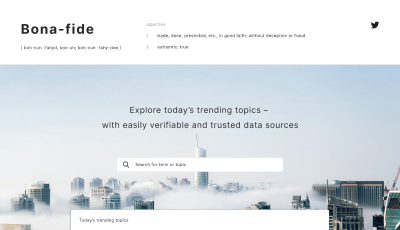A screenshot of a website showcasing the brand "BonaFide" is captured in this image. In the top left corner, prominently displayed in black text, is the logo "Bona-Fide." On the top right corner, a black Twitter logo is visible. Between these elements, there is some text that resembles a dictionary definition, though it's too small to be clearly read. Dominating the background, a large image depicts a futuristic cityscape with skyscrapers emerging through a blanket of clouds. Central to the layout is the tagline: "Explore today's trending topics with easily verifiable and trusted data sources." Below this, a conspicuous white search bar invites user interaction. Further down, the section labeled "Today's Trending Topics" adds a touch of engagement. The caption concludes with a courteous sign-off: "Thank you for watching."